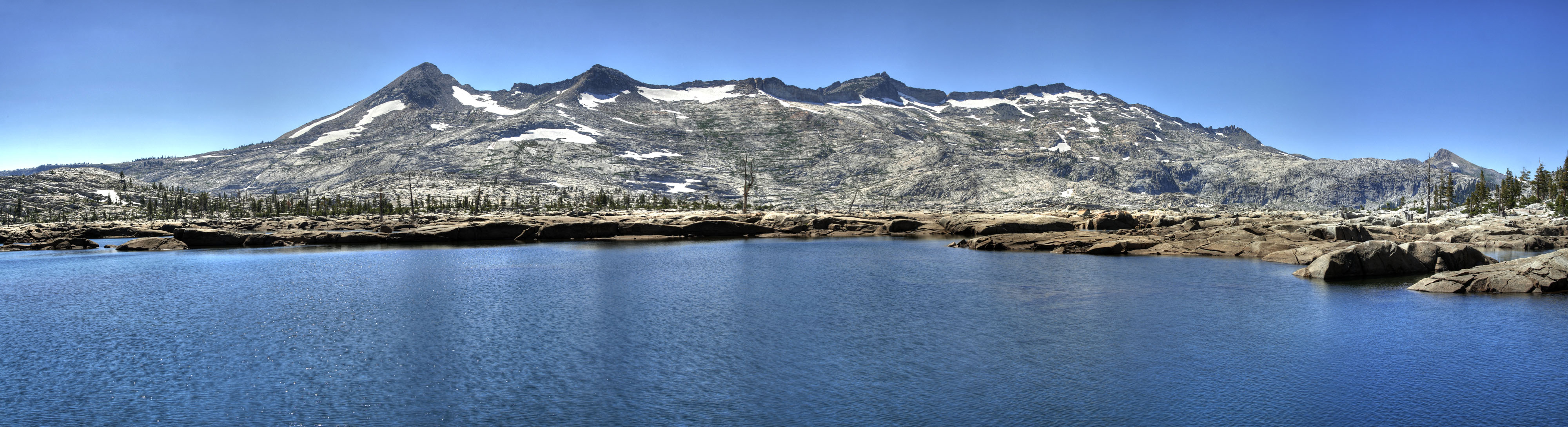A stunning, panoramic outdoor scene captures the serene beauty of a mountainous landscape during daytime. The image, with a wider than tall aspect ratio reminiscent of a web banner, showcases a crystal-clear, tranquil mountain lake at the bottom, bordered by a rocky shore composed of large stones. To the left and right of the lake, a sparse yet increasingly prominent row of pine trees adds a touch of verdant green to the landscape.

In the background, dramatic, craggy mountains loom, their gray rocks contrasted by darker peaks and topped with snow, suggesting either the winter season or a high-altitude location, possibly somewhere in Wyoming. The deep blue sky gradually darkens towards the top right corner, adding depth and a sense of vastness to the image.

Absent of people and animals, the scene exudes tranquility and natural beauty, making it a captivating and pristine snapshot of nature's splendor.